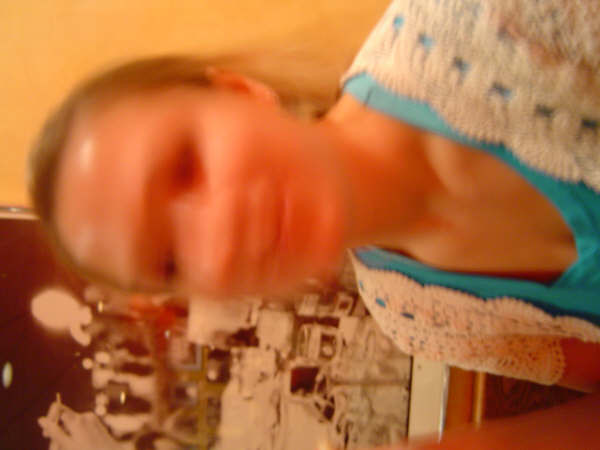A very blurry photograph captures a woman rotated sideways, requiring a 90-degree clockwise rotation to be viewed properly. The woman, likely in her mid-20s with light brown hair pulled back in a ponytail, wears a green t-shirt material blouse with a low plunging neck, over which she has a white, crochet-style woolen cardigan. Her face is largely indecipherable due to the blur, making her facial features almost unrecognizable, and lending a somewhat eerie quality to her appearance. She appears to be sitting in front of a yellow background, partially obscured by a large, dark-framed painting with indistinct white designs, possibly depicting computer components. There’s also a suggestion of a reddish tint to her face, and nearby objects like what could be glasses. The overall scene is both perplexing and intriguing due to the blurry, sideways nature of the image and the unclear background elements.